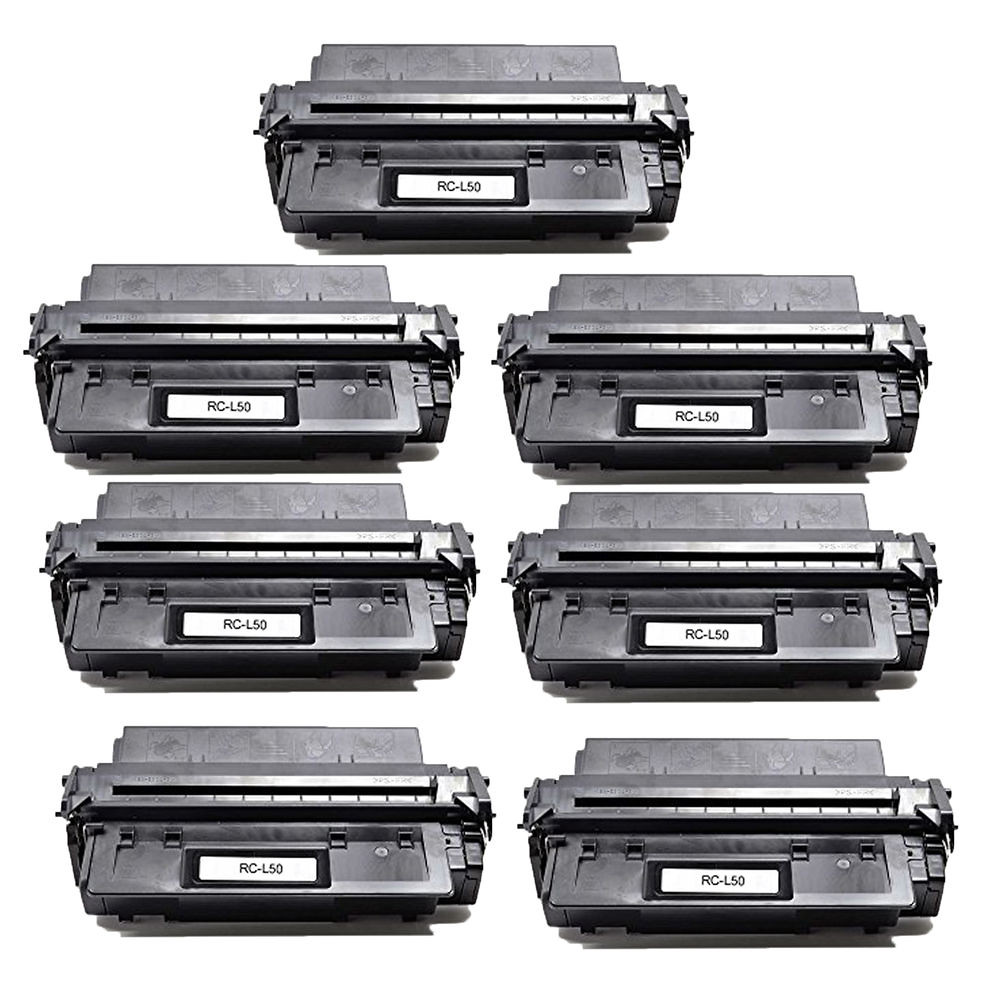This black-and-white image features seven identical machines that resemble printers or word processors, each labeled with "RC-L50" on an LCD screen located toward the middle-front of the devices. The image is set against a transparent background, and each machine has a consistent dark gray-black color scheme. Six of these are arranged in two rows of three, and one additional device is positioned above the rows, centered. All machines have a raised separator feature, likely for paper handling. The photo focuses solely on these devices, cropped out of any specific environment, emphasizing their uniformity and design.